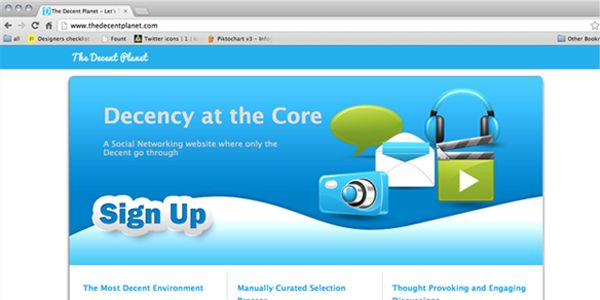The image features a website interface with a prominent, long gray search bar at the top. Below the search bar, there is a white field displaying the URL "www.thedecentplanet.com." Beneath this is a long blue banner with the text "The Decent Planet" written in white cursive.

Centered on the page is a large rectangular box, roughly four inches wide by five inches tall. The box has a background that transitions from dark blue at the top to light blue at the bottom. Inside this box, white text reads: "Decency at the Core - A social networking website where only the decent go through." Below this statement, there is a sign-up button with "Sign Up" written in blue, bubble letters.

To the right of the text box are several icons: a green speech bubble, a blue camera, a white envelope with a small blue piece of paper inside, blue headphones with black ear pads, and a film clapperboard. The top of the clapperboard is black and gray, while the bottom is green with a white play arrow.

At the bottom left corner, blue text reads: "The most decent environment." Just below this is another blue text: "Manually curated selection." In the bottom right corner, more blue text declares: "Thought-provoking and engaging."